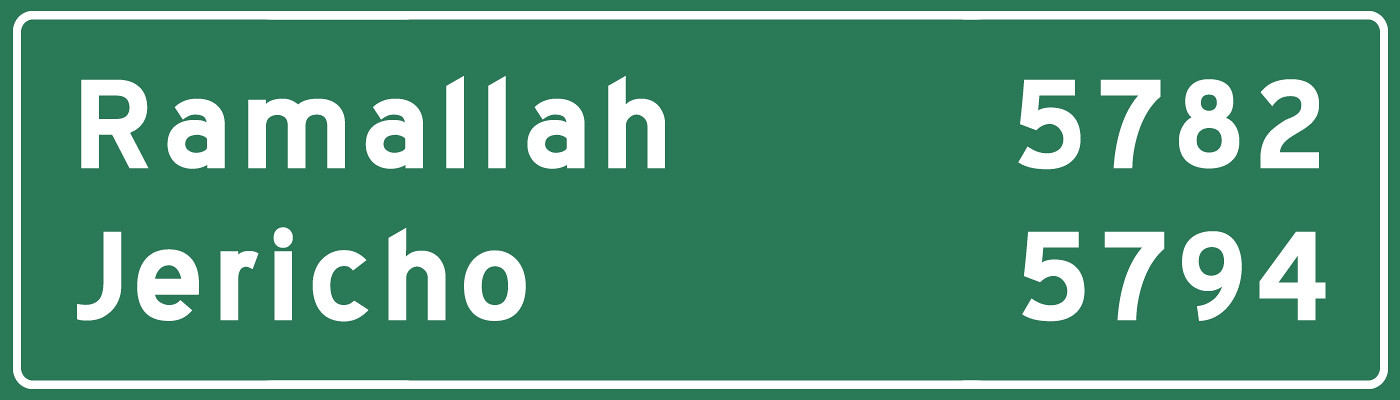The image showcases a horizontally long, green highway sign with a white border and a thin green outline around the edges. The white text on the sign prominently features the destinations and distance figures: on the top left, "Ramallah" is written with the number "5782" to its right, indicating either distance or some other metric. Below that, "Jericho" is noted, followed by the number "5794." The sign is designed to guide travelers to the cities of Ramallah and Jericho.